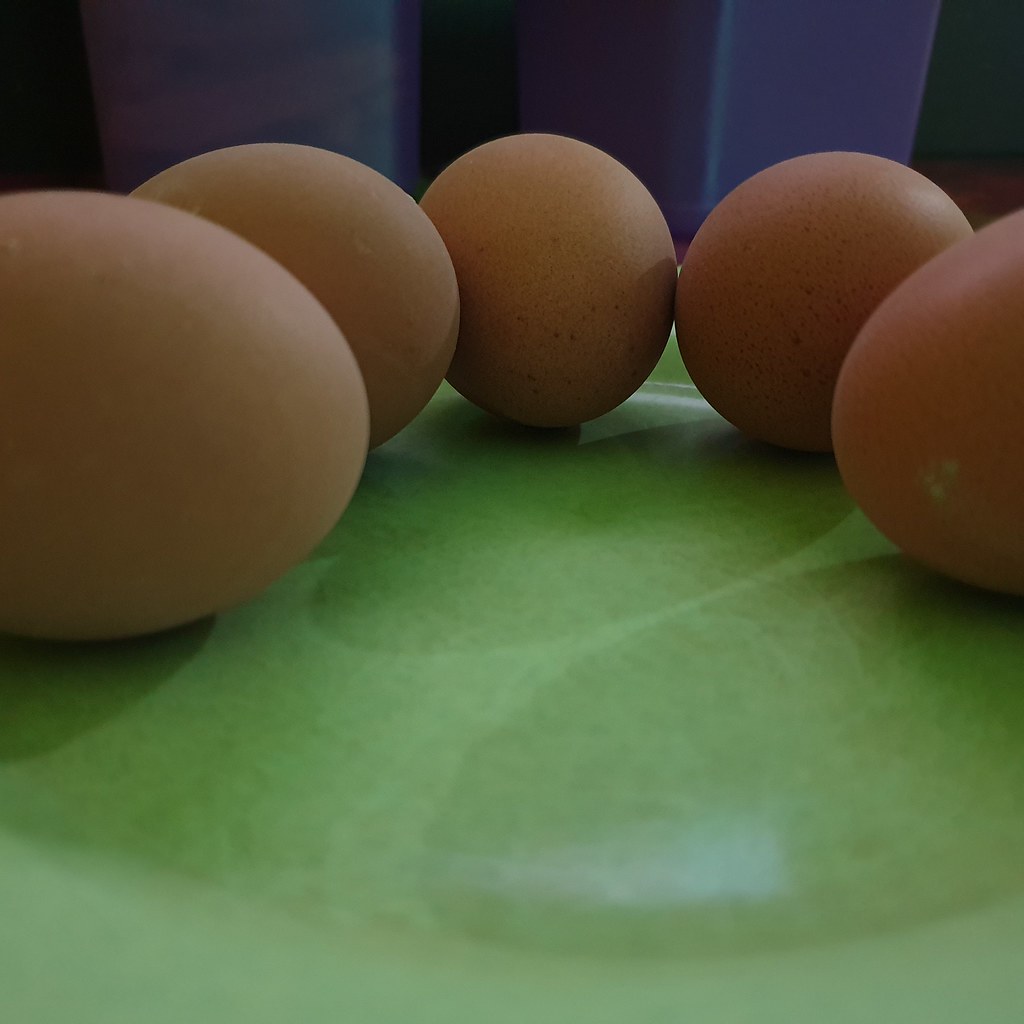This close-up square photograph captures five large, naturally colored eggs arranged in a semicircle on a jade-colored, green surface that resembles marble. The eggs, varying from light brown to a darker reddish-brown, have stains and speckles on their shells. The eggs cast distinct oval shadows on the surface, enhancing their natural appearance. The backdrop features a deep purple, curtain-like background with vertical ridges. The image tightly focuses on the eggs and the green surface, providing a detailed and intimate view of the scene.